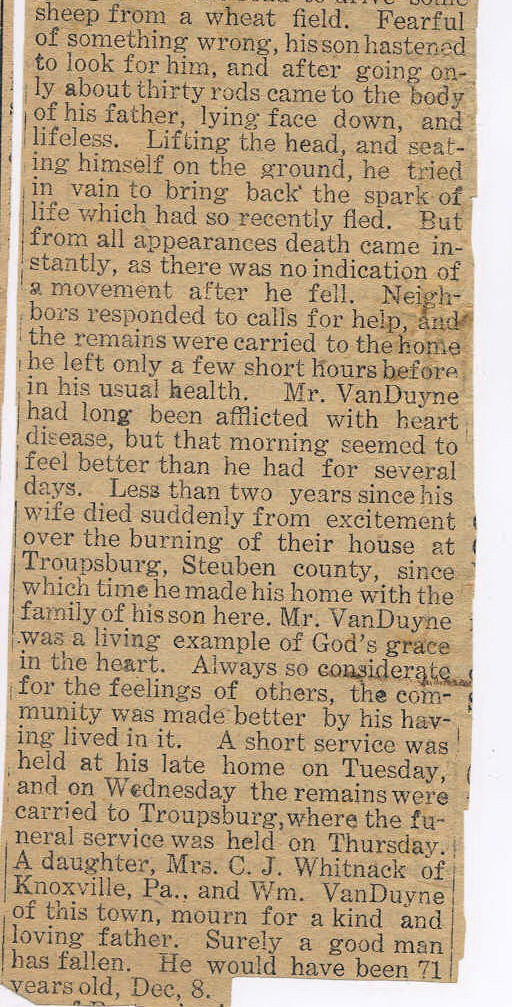This image is a fragment of an old newspaper clipping, carefully cut out in a vertical segment, with no title and abruptly ending midway through a sentence. The brownish hue of the paper and black inked text hint at its age. The passage, incomplete due to the asymmetric cut at the bottom, starts in the middle of a sentence: "Sheep from a wheat field, fearful of something wrong, hissed and hastened to look for him. And after going only about thirty rods, came to the body of Mr. Van Dine, lying face down and lifeless. Lifting the head and seating himself on the ground, he tried in vain to bring back the spark of life which had so recently fled. But from all appearances, death came instantly as there was no indication of a movement after he fell. Neighbors responded to calls for help, and the remains were carried to the home he left only a few short hours before in his usual health." 

The article continues to describe that Mr. Van Dine had long suffered from heart disease but felt unusually well that morning. It mentions that less than two years prior, his wife passed away suddenly due to excitement over a house fire. Dr. Van Dine had since lived with his son’s family. The article commends Mr. Van Dine as a paragon of godliness and community spirit, and recounts the grief of his children, Ms. C.J. Whitnack of Knoxville, Pennsylvania, and W.M. Van Dine. It notes that a short service was held at his late home, followed by a funeral service in Troopsburg. Mr. Van Dine would have been 71 years old on December 8th.